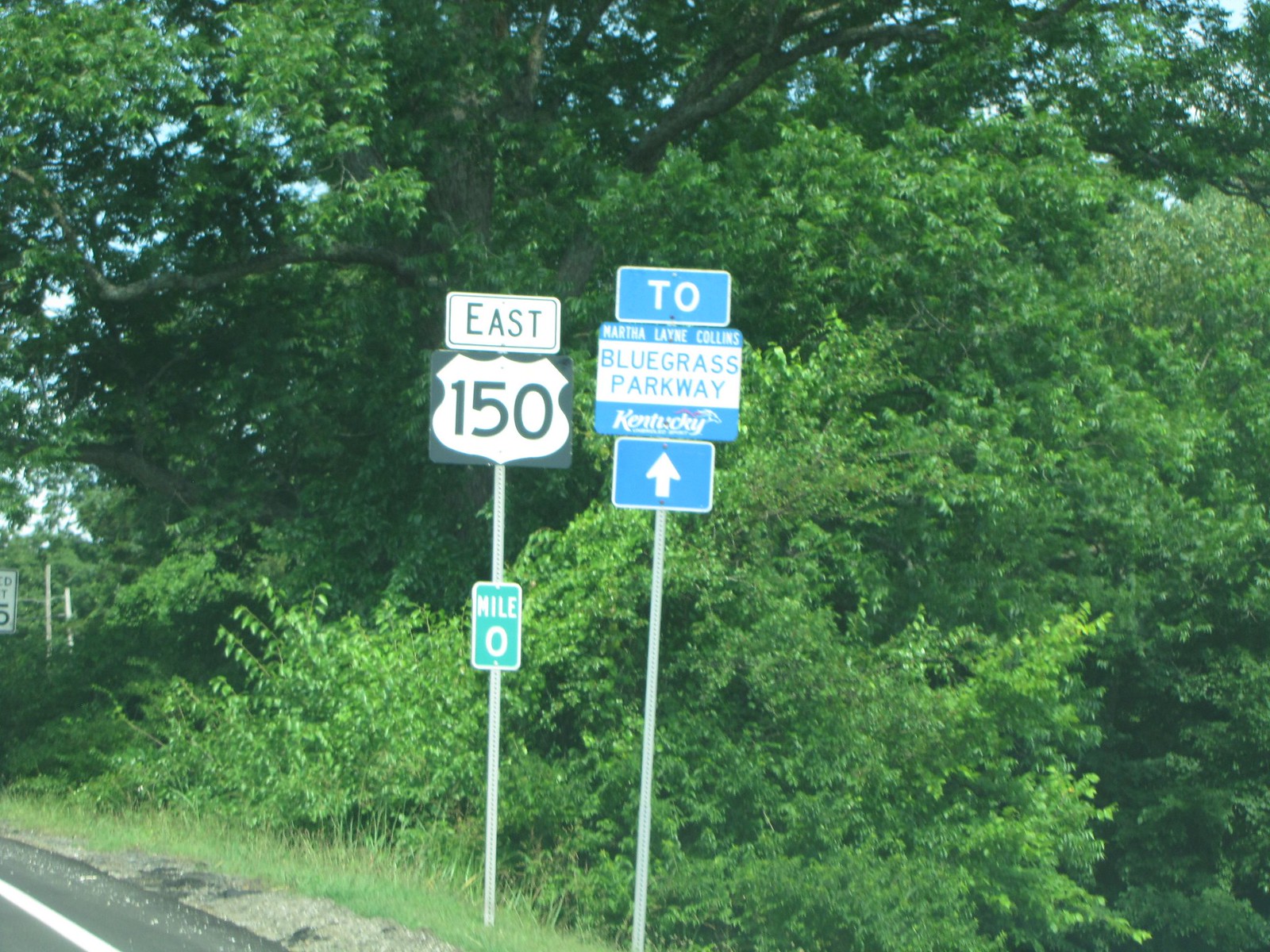This outdoor photograph captures a lush, verdant roadside scene, dominated by various shades of green from dense trees and bushes that provide a natural backdrop. Patches of blue sky peek through the foliage, especially noticeable at the top and left of the image. The lower left corner showcases a portion of the roadway, where a white line marking the right side of the street is visible.

Prominently positioned in the middle of the image are two traffic signs erected on metal posts. The sign on the left features a rectangular sign at the top with "EAST" inscribed in black letters. Beneath this, a highway sign displays the number "150" on a white background encased within a black rectangle. Further down, a green vertical rectangular sign indicates "MILE 0" in silver letters.

The sign on the right consists of a series of blue and white components. At the bottom, there's a blue rectangular sign adorned with a white arrow pointing upward. Directly above it is a white rectangular sign with "BLUEGRASS PARKWAY" written in blue capital letters. This is flanked by blue bands above and below, carrying additional text in white letters on a blue background. Crowning this sign is a horizontal blue rectangle labeled "TO" in white capital letters.